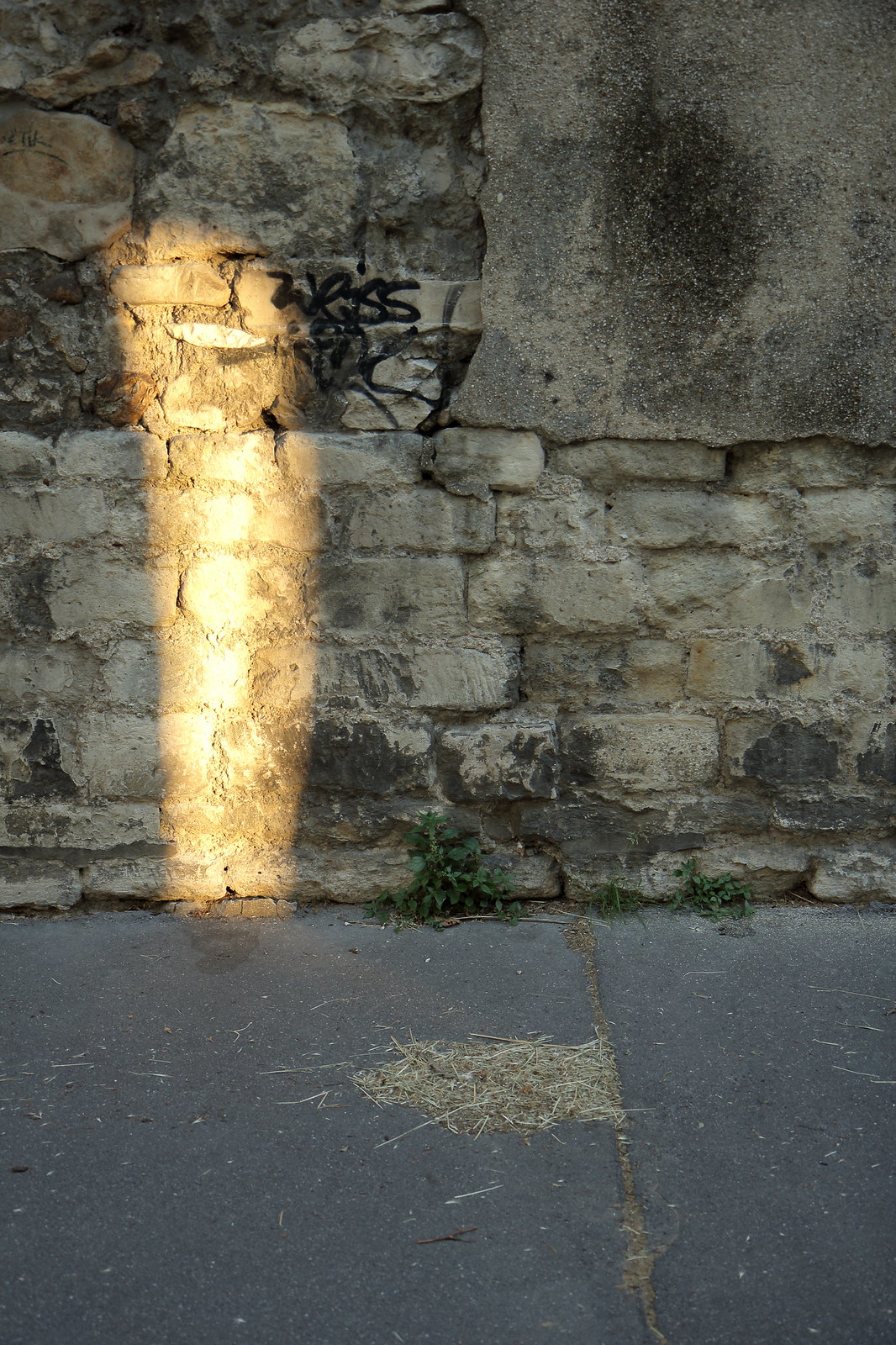The image showcases a dark gray concrete sidewalk adjacent to a rugged, multi-hued stone wall in shades of beige, gray, and brown. Along the sidewalk lies a pile of straw or dried grass, enhancing the rustic feel of the scene. Weeds and small green plants sprout at the base of the wall, lending a touch of nature amid the urban environment. The stone wall, which appears to have once been covered in mortar now flaking off, features black graffiti with the writing "WESS" and additional initials below it. A striking beam of sunlight creates a nearly ghost-like vertical line on the left side of the wall, adding a dramatic element to the photograph. The overall scene suggests a contemporary, well-maintained environment despite the worn appearance of the wall.